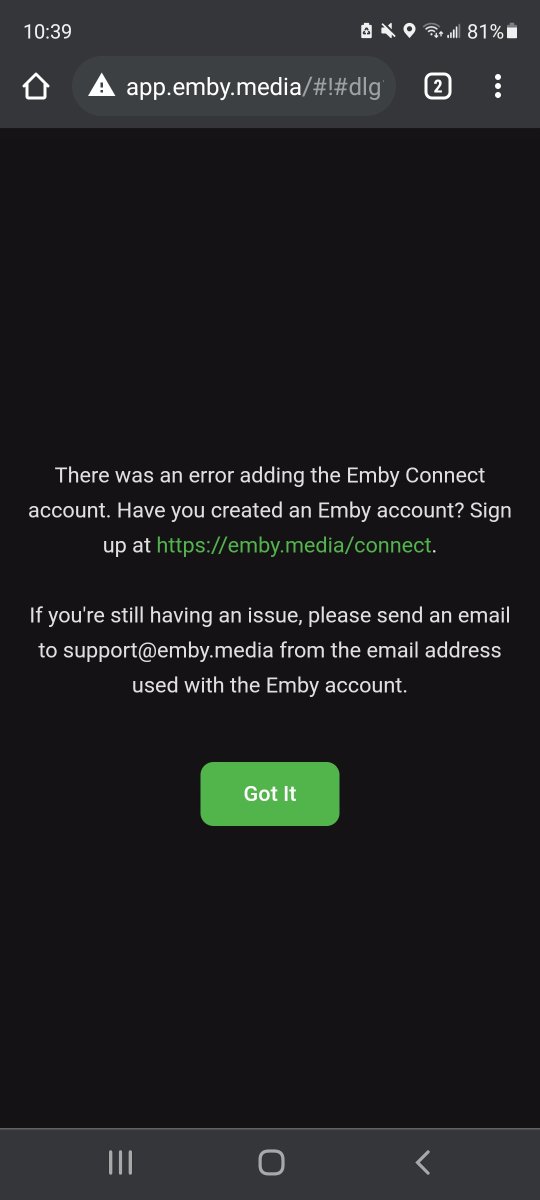The screenshot displays a mobile phone interface with a light charcoal status bar at the top, showing the time (10:39), battery life (81%), and icons including an upward arrow and white warning triangle. The bar also contains the text "app.mb.media" and an icon with three dots for more options.

The main section of the screen features a black background. Near the top center, in white text, there is a message stating, "There was an error adding the MB Connect account." Below that, a prompt inquires whether you have created an MB account and suggests signing up at a URL depicted in dark green text: "https://mb.media/connect." Further instructions in white text recommend sending an email to "support@mb.media" from the associated MB account email if issues persist. 

At the bottom of the screen, a prominent lime-green button with white lettering reads "Got it." Below this button, the standard phone navigation icons (such as back, home, and recent apps) are visible.